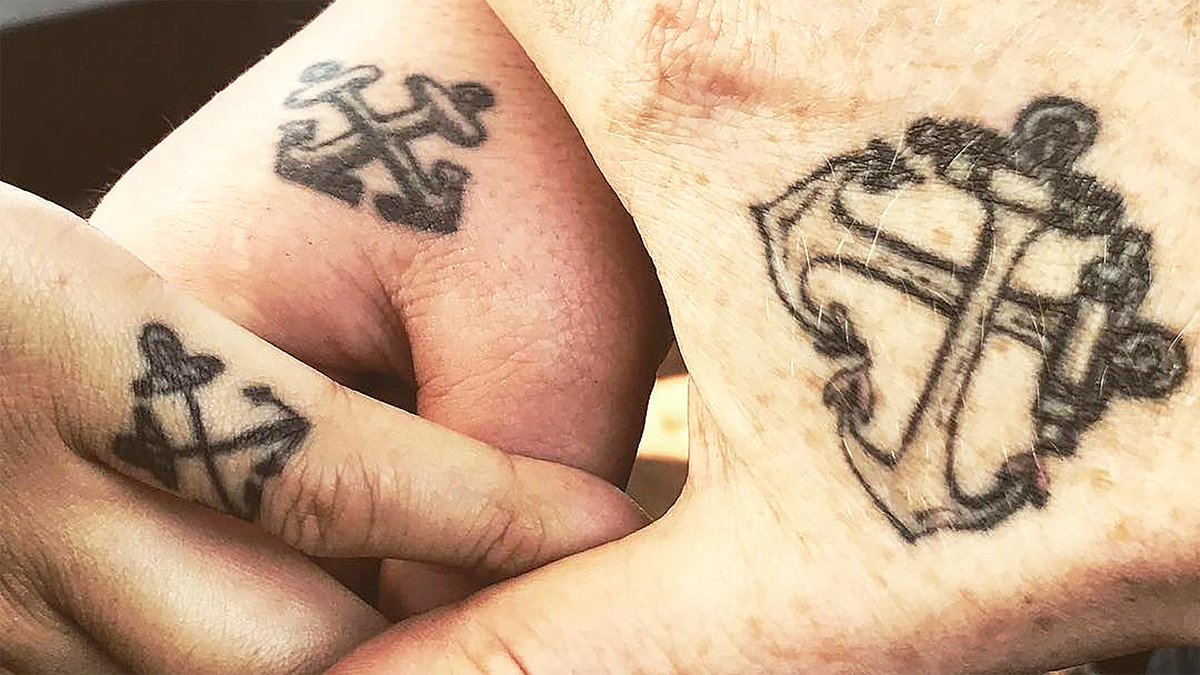This up-close color photograph displays three different hands, each showcasing a black ink tattoo of two crisscrossed boat anchors. The hand on the right side is notable for its lighter complexion with freckles, featuring the tattoo prominently between the thumb and index finger near the thumb's base. In the middle of the image, another hand presents a similar tattoo in the webbing between the thumb and index finger. The hand in the lower left corner displays its tattoo along the index finger, positioned between the third and second knuckle. The recurring theme of crisscrossed boat anchors unites the intricate designs across all three hands.